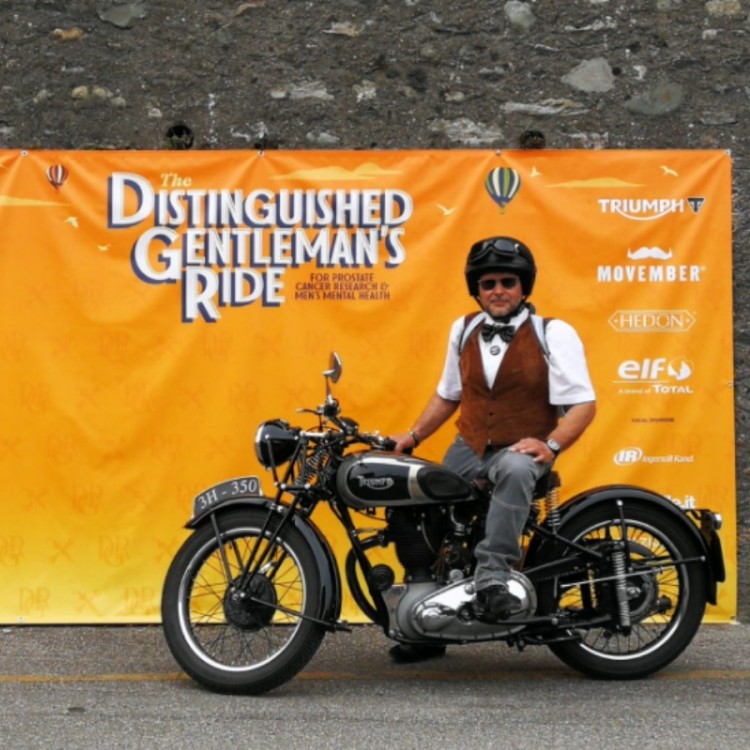The photograph captures a man sitting on a silver and black Triumph motorcycle, which is oriented to the left. The left side of the motorcycle is visible, with specific details such as a silver-trimmed black tank featuring the Triumph logo and a round black headlight with a silver border. The front wheel displays the numbers "3H350" near the headlight, likely indicating a license plate.

The man is dressed in a white short-sleeved collared shirt paired with a chocolate brown vest and a black bow tie. He has gray slacks and black shoes on. For safety, he’s wearing a black helmet, and he also has dark sunglasses on, with goggles resting atop the helmet. There are straps over his shoulders, possibly indicating a backpack. A wristwatch adorns his left wrist, which is placed on his left knee, while his right hand rests on the motorcycle’s body.

Behind him, an expansive orange banner with a stone wall above it adds context to the scene. The banner prominently features "The Distinguished Gentleman's Ride" in white text on the upper left side, alongside smaller blue writing. It continues to the right with logos for sponsors including Triumph, Movember, Hedon, Elf, Total, and IR, promoting causes like prostate cancer research and men’s mental health. The road beneath the motorcycle is asphalt, transitioning to a background of mud and rocks beyond the banner's edge.